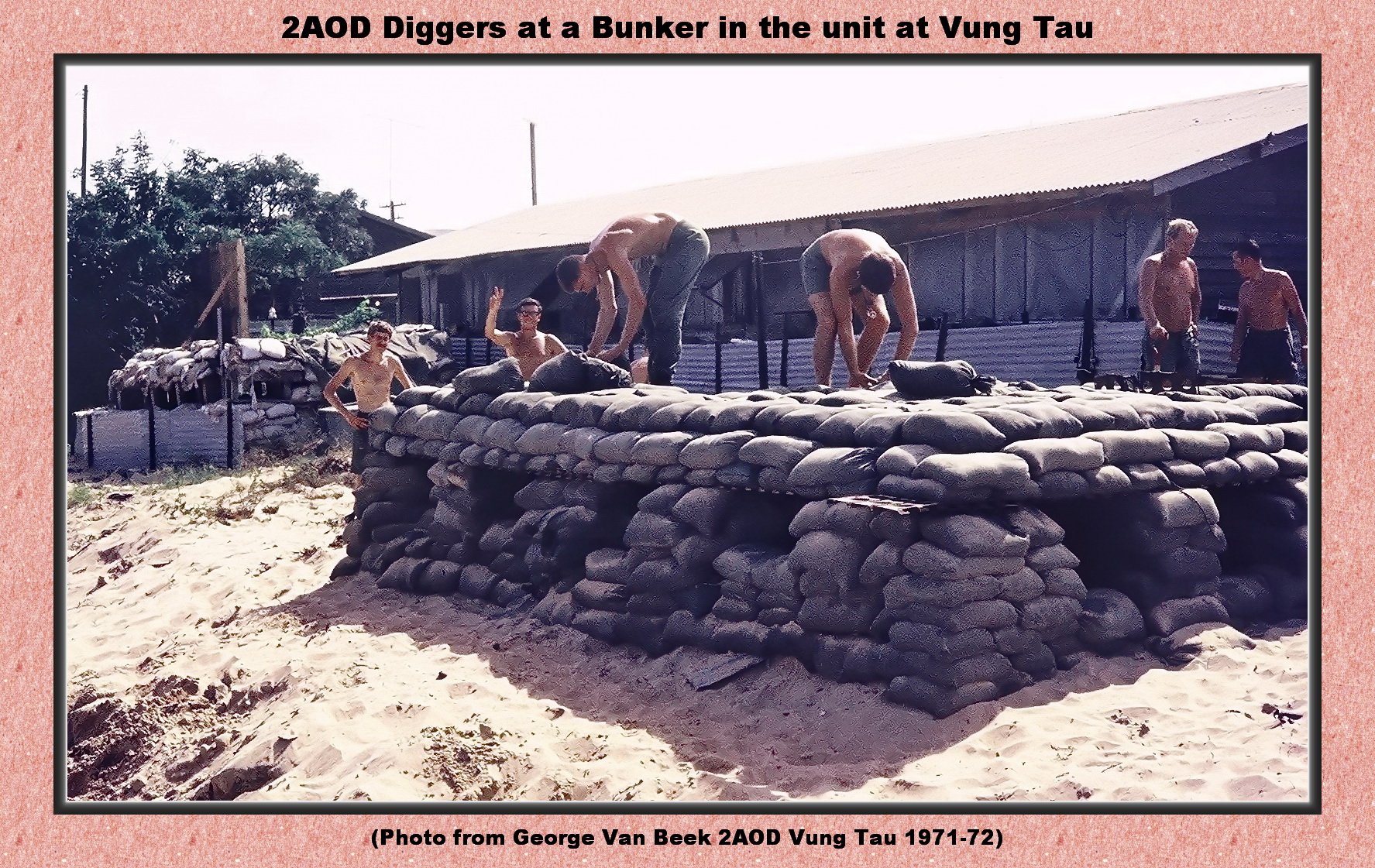The photograph depicts six shirtless U.S. soldiers in army pants constructing a four-foot-tall bunker using dark sandbags. They are organized with three men on the left, one in the center, and two on the right. The background showcases a metal building with a corrugated roof, reflecting a light brownish tint, possibly from the sun. The bunker features square holes designed for visibility and defense. The setting appears to be at a beach, indicated by the sand below and around the soldiers. The photograph includes two captions: above the image, it reads, "To AOD, diggers at a bunker in the unit at Vung Tau." Below, it states in parentheses, "Photo from George Van Beek. To AOD, Vung Tau, 1971-72." The entire image is in color.